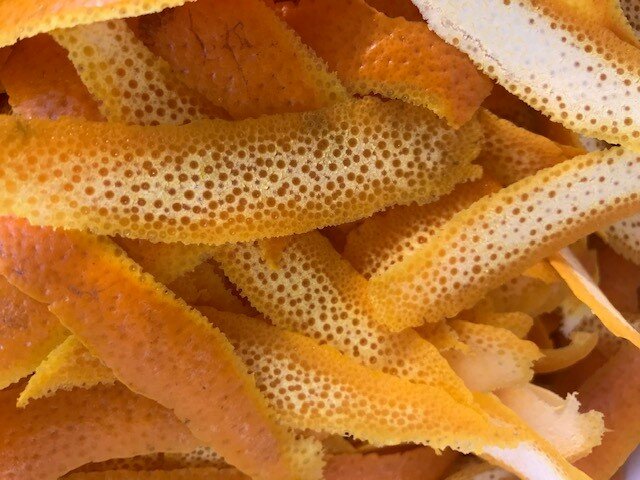This is a detailed close-up image of a large pile of orange zest, consisting of long, narrow strips of orange peel. The peels are in various orientations, scattered and piled atop one another. The exterior side of many strips showcases a shiny, dark orange color, while the underside reveals a lighter orange to almost white hue, often dotted with small circular indents. These details suggest that care was taken to avoid the bitter part of the peel. Notably, in the top right corner, there are a couple of strips that are predominantly white on the inside. The image captures the varied texture and color differences between the outer and inner layers of the orange zest, presenting an intricate and vibrant composition of orange peelings.